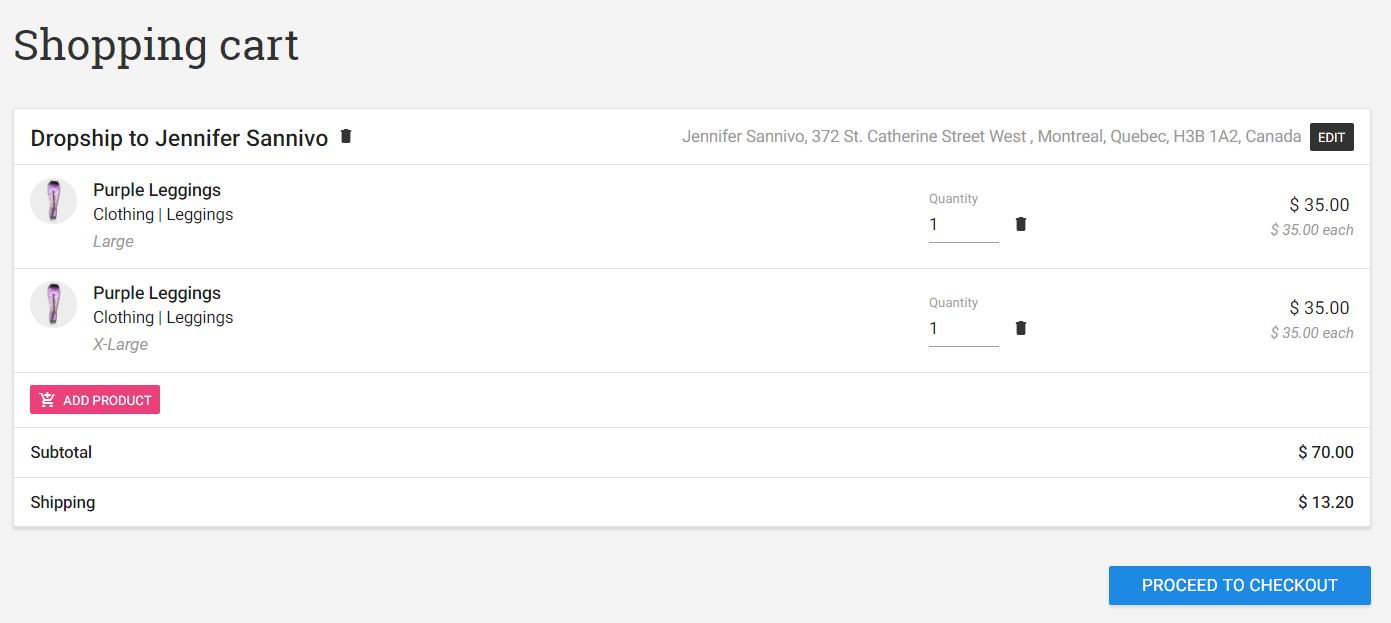In the shopping cart screen capture, there are two pairs of purple leggings listed. The items are categorized as "clothing/leggings," with one pair labeled as size large and the other as extra large. Each listing features a small circular profile image showcasing a person wearing the purple leggings. The customer is identified as Jennifer Sanovo, with a shipping address of 372 St. Catherine Street West, Montreal, Quebec, H3B 1A2, Canada. 

A quantity of one is displayed next to each item, alongside a black trash can icon that allows for deletion. The cost of each pair of leggings is $35, accumulating to a subtotal of $70. Additional shipping charges amount to $13.20. Overall, the detailed interface includes an option to edit the order and a prominent blue "Proceed to Checkout" button at the bottom.